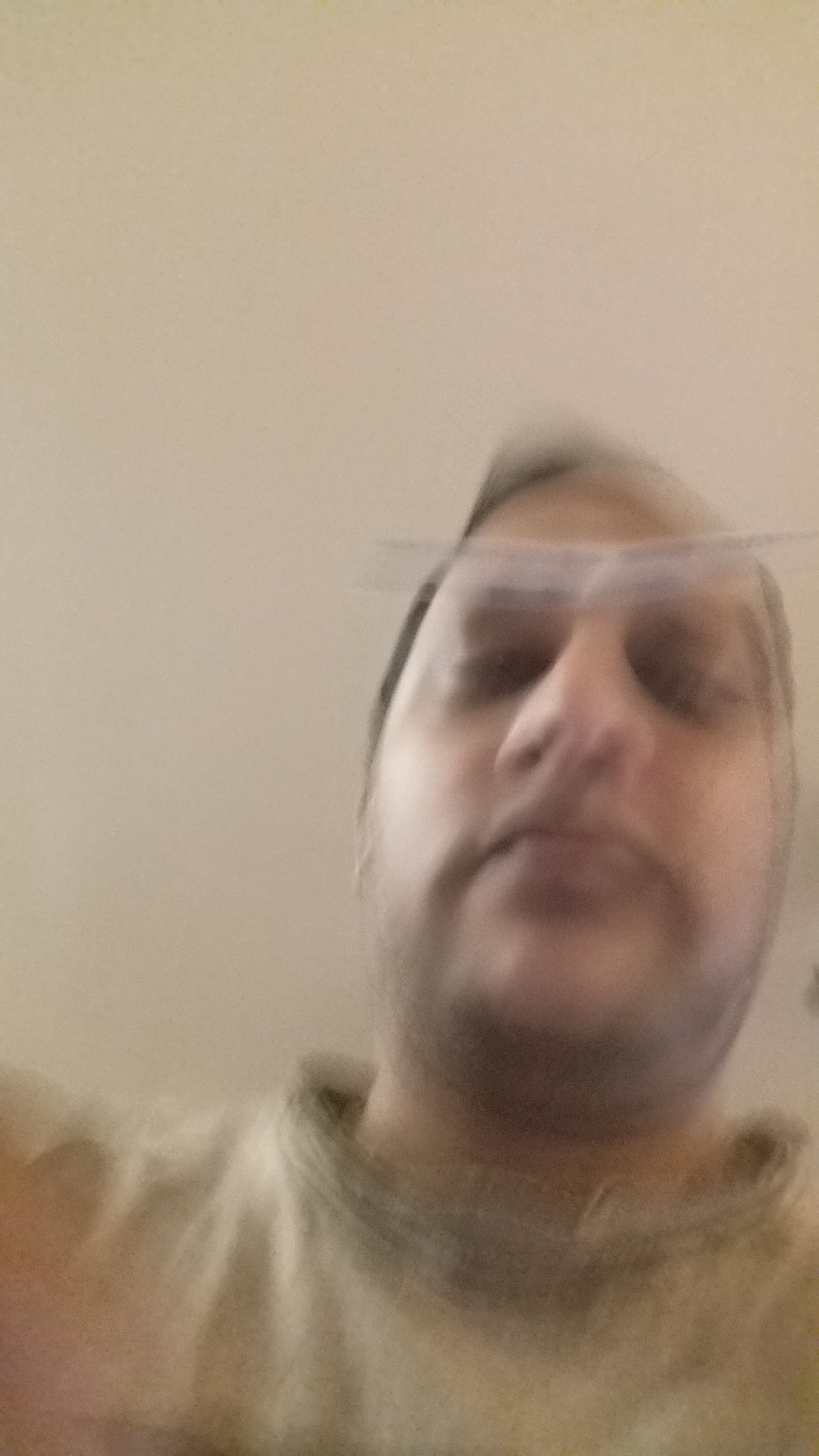This image is an extremely blurry selfie of a man with light brown skin. The photograph appears to be taken indoors, as indicated by the beige ceiling in the background. The man is possibly in motion, contributing to the blurriness, and his hand is visible in the bottom left, also appearing to move. He has thin black hair and a fuzzy beard, giving him a five o'clock shadow look. He is looking down at the camera, which is angled upward towards him. He has a large, rounded nose and full lips that form a slight frown, giving his expression a somewhat somber appearance. His eyes are lowered, suggesting he might be trying to read something on the phone. He is wearing glasses positioned at the top of his eyebrows, and he is dressed in a light green turtleneck, with the collar and part of the right shoulder visible. The overall setting implies he is inside a building.